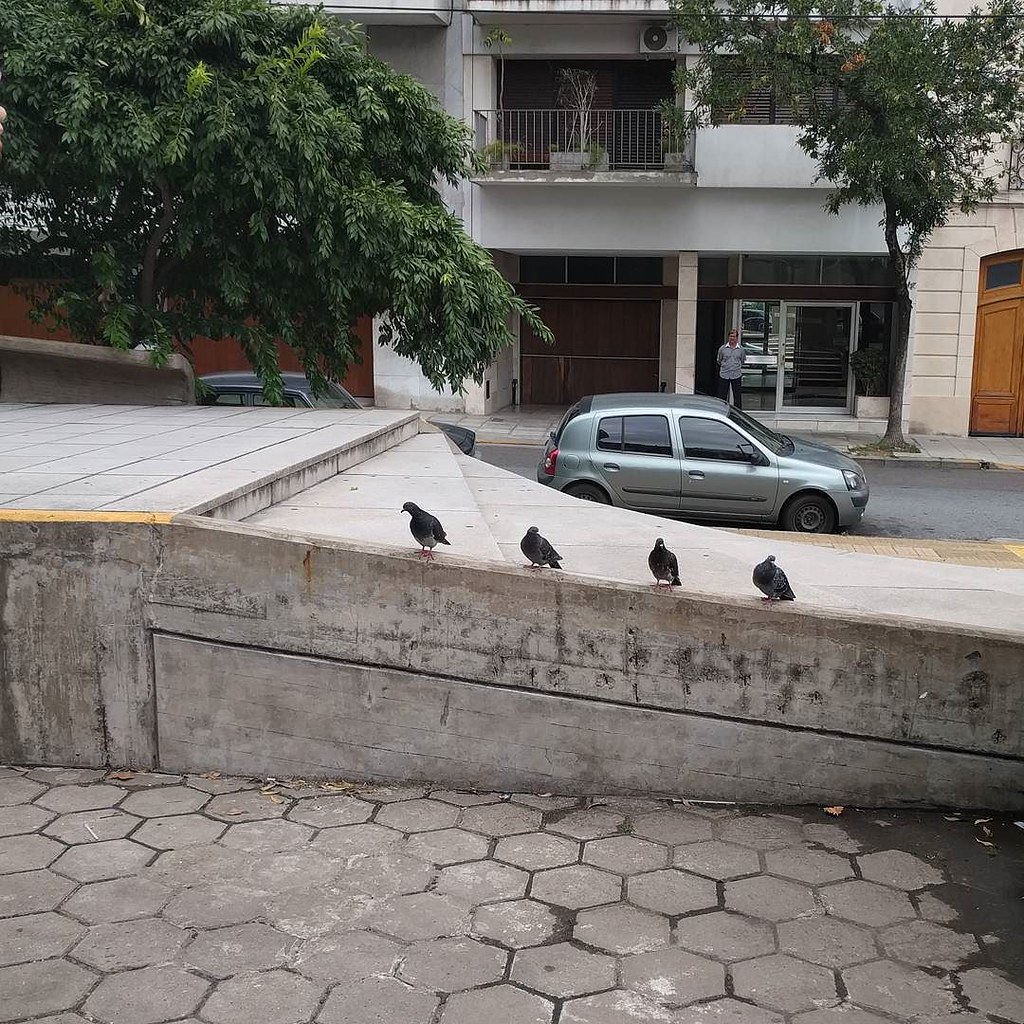A bustling city street scene features a sidewalk bordered by a concrete barrier, beyond which lies a road. Standing prominently on the concrete barrier are four crows, each with sleek black feathers, appearing contemplative as they observe the surroundings. Behind the crows, a set of slightly spiral stairs ascends to a platform that exits the frame to the left. A blue four-door car is parked with its front end facing right and its back end toward the left, accompanied by the roof of a black car and a tree with lush green leaves occupying the upper right corner. Overlooking the scene is a gray, two-story apartment building with a balcony on the top floor adorned with a fence and plants. On the ground level, the building features brown doors with windows and a glass door framed by brown trim. Nearby stands a person with a white collar, blue shirt, and black pants, adding a touch of daily life to the urban tableau.